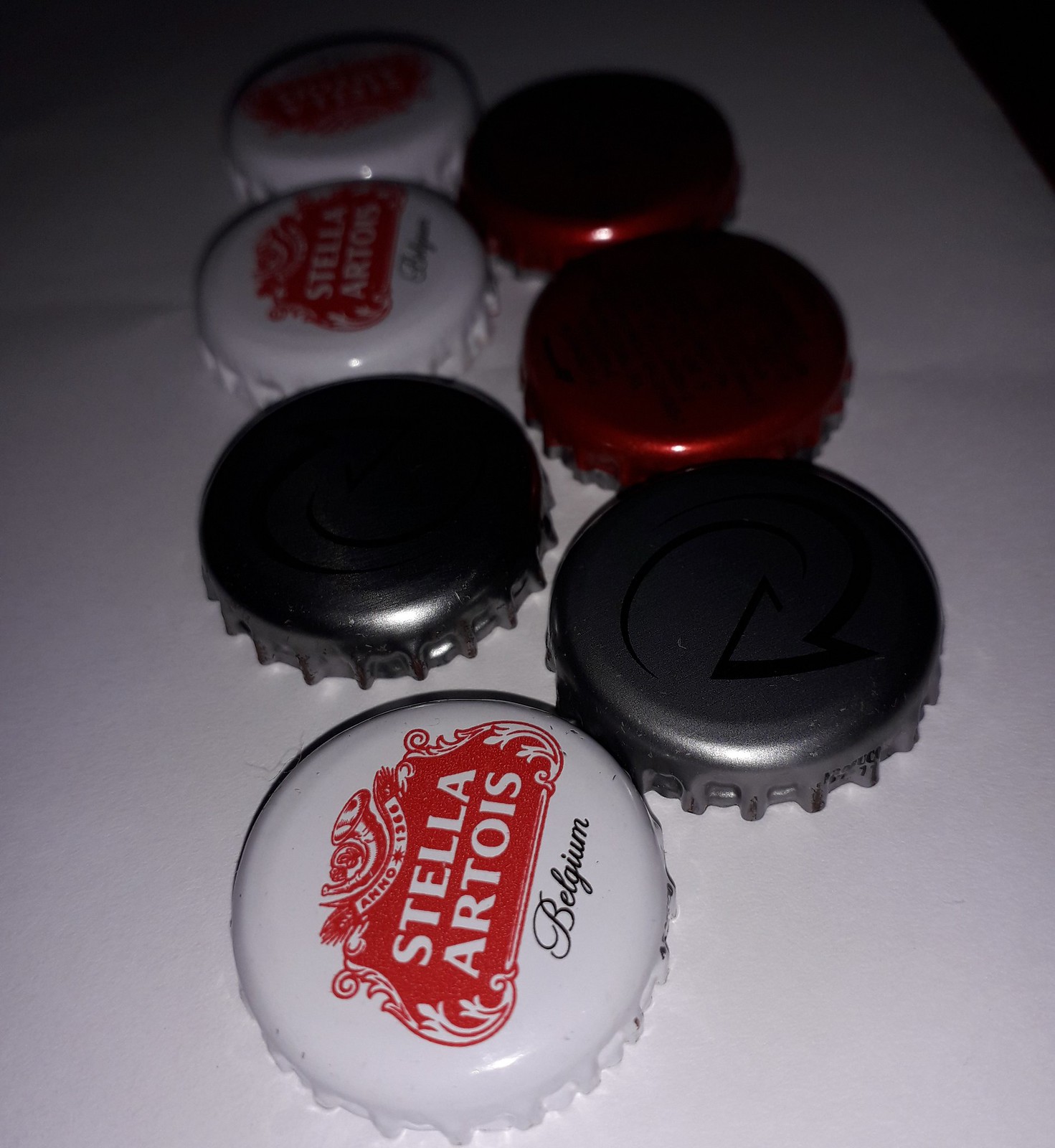This photograph showcases seven beer bottle caps arranged in a staggered, zipper-like pattern on a white surface, primarily illuminated by the camera's flash. The left column consists of four bottle caps: from top to bottom, three are white with the red Stella Artois logo and "Belgium" written underneath, and the fourth is a dark silver, nearly black cap. The right column contains three caps: the top two are dark red, but their logos are obscured by shadows, and the bottom one is a dark silver cap similar to the one on the left. The overall image is quite shadowed, highlighting the contrast between the brightly lit caps and the darker surroundings.